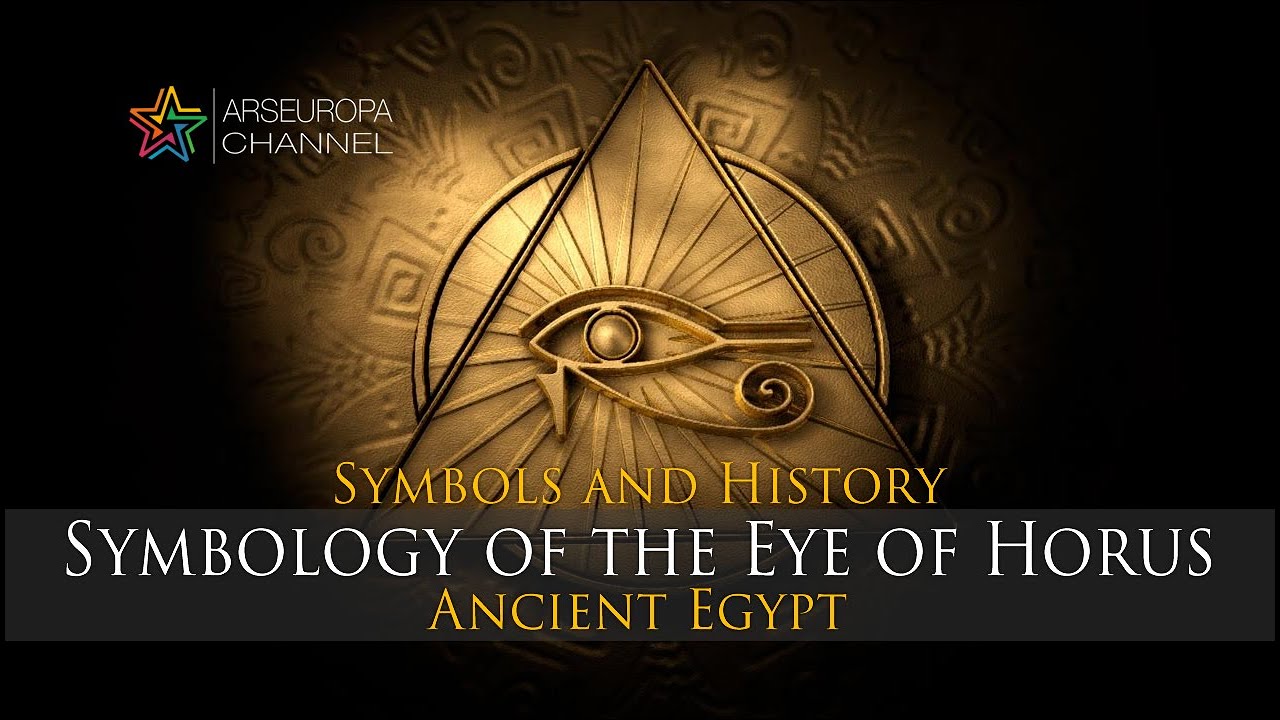The image features a wide, black rectangular background resembling a TV show screenshot or an advertisement. In the top left corner, there's a vibrant multicolored star logo with shades of yellow, green, blue, violet, red, and orange. Below the star, the text "R.C. Ars Europa Channel" is prominently displayed. Central to the image is a golden pyramid with a detailed Eye of Horus at its peak, encircled by beams of light and surrounded by intricate Egyptian hieroglyphic symbols. Beneath this central image, the caption "Symbols in History" appears in yellow, followed by "Symbology of the Eye of Horus" in white, and "Ancient Egypt" in yellow. The overall design integrates additional dark gray tones to enhance its mystical and historical theme, suggesting content related to Ancient Egyptian artifacts and their symbolism.